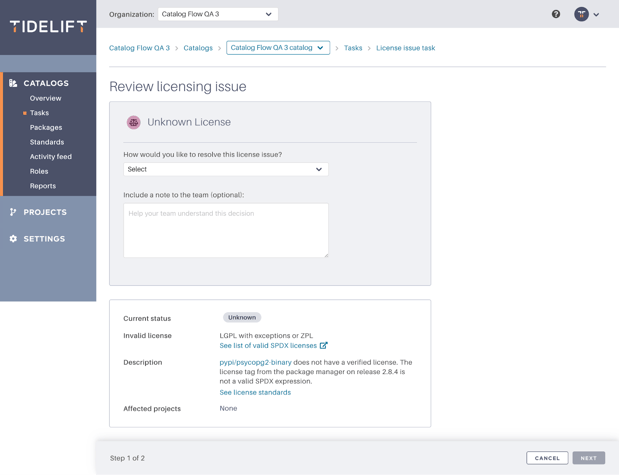This image is a detailed screenshot of the Tidelift website, a service aimed at developing or maintaining websites and web applications, catering primarily to programmers. In the image, the Tidelift logo is prominently displayed in the top left corner, featuring stylized 'T's that transition from white at the top to orange at the bottom. Directly beneath the logo, there is a vertical navigation menu housed in a blue box, listing options such as "Catalogs," "Projects," and "Settings."

The central portion of the screenshot features the main workspace of the Tidelift interface, highlighted by a predominantly white background interspersed with light gray boxes. The focal point of this section is the "Review Licensing Issue" page, as indicated by the prominent black text heading. A gray box below this heading declares "Unknown License," and provides additional information to guide the user on resolving the identified licensing issue.

At the bottom of the main page, detailed information is laid out in a scheme combining black text with a white and gray background. This section includes specifics about the current license status, which is flagged as invalid, along with a description and the names of affected projects. The page indicates that this is "Step 1 of 2" in the process of correcting the issue, as stated within a gray horizontal bar at the bottom center.

Finally, two actionable buttons are located at the lower right: a "Cancel" button, styled with gray text on a white background, and a "Next" button, distinguished by white text on a dark gray box.